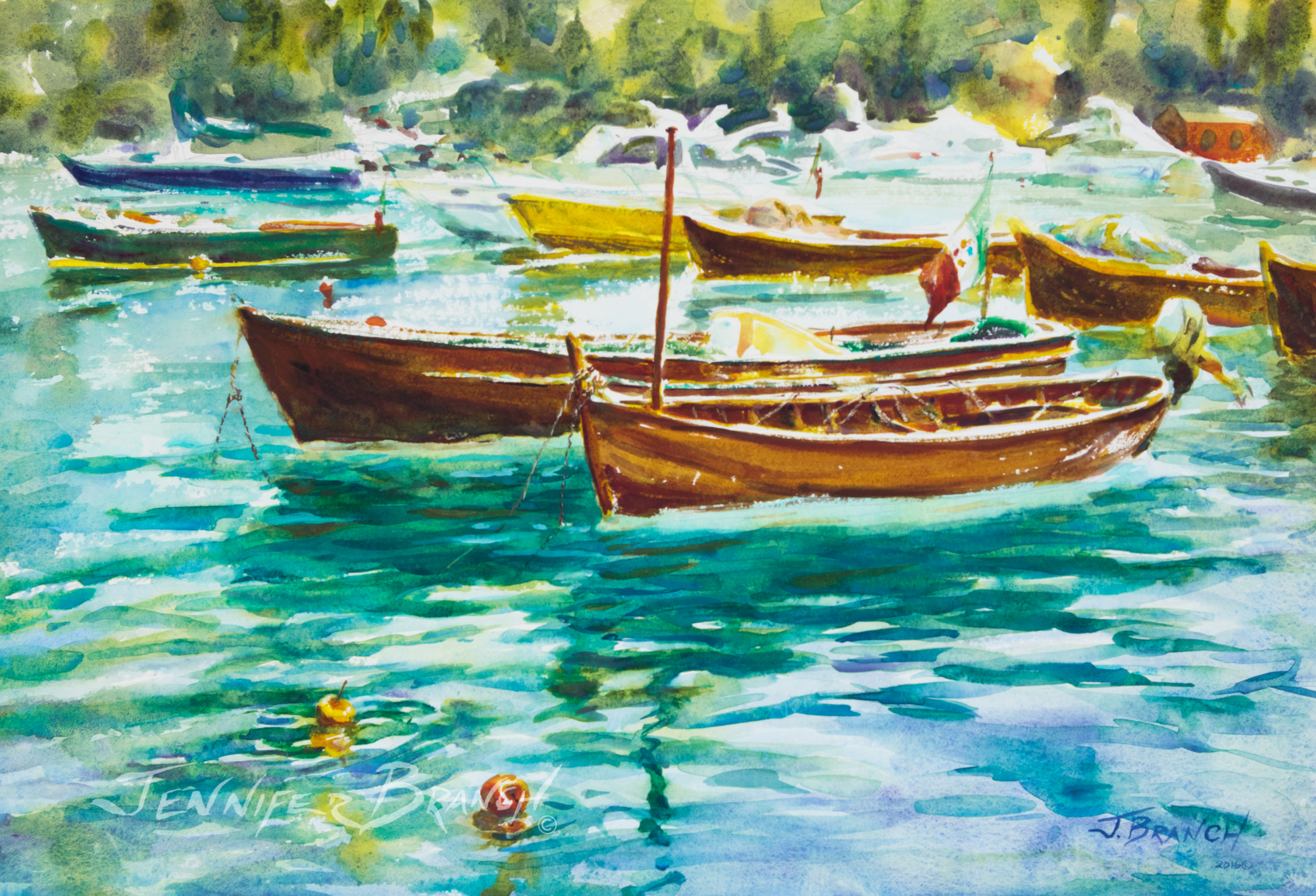The painting signed by Jay Branch on the bottom right corner and Jennifer Branch in white watercolor lettering across the bottom left corner, is a beautiful and impressionistic piece created in 2016. It depicts approximately eight to nine wooden rowboats or canoes of various tones, including brown, green, and yellow, moored serenely on a reflective water surface, which is beautifully rendered with a harmonious palette of greens, blues, purples, and hints of lime green and yellow. The water, dotted with floating apples in the far bottom left-hand corner, shimmers under an array of vibrant colors, suggesting a peaceful and idyllic setting. In the backdrop, the painting features a shoreline embellished with impressionistic trees and foliage, with indistinct yellows, greens, and blues hinting at a lush natural environment. A small cabin is discernible amidst this foliage, offering a quaint accent to the scene. A flag, possibly resembling the Mexican flag, adorns one of the boats, adding a touch of detail to the tranquil tableau. The entire scene exudes a soft, almost dreamy quality characteristic of the impressionistic style, leaving the viewer with a sense of serenity and calm.